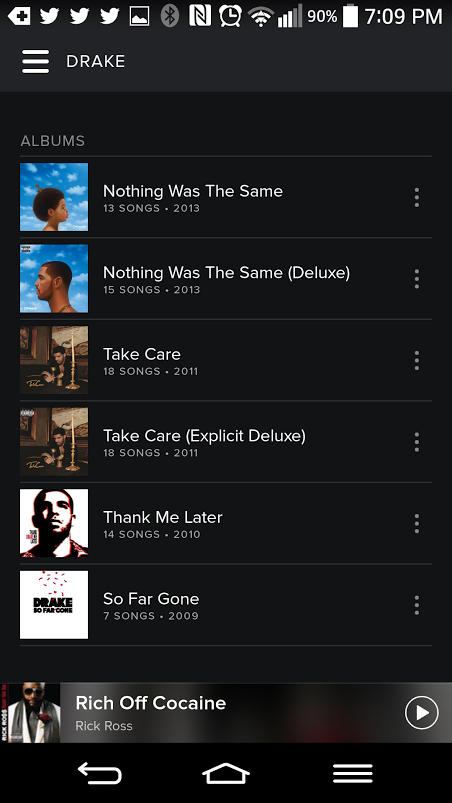A detailed screenshot of a cell phone with a completely black background. The top of the screen displays various status bar icons, starting from the left: a plus sign, three Twitter bird icons, an image icon, a grayed-out Bluetooth symbol, an 'end' sign, a clock icon showing the time as 7:09 PM, a Wi-Fi signal icon, a data connection symbol, '90%' indicating battery level, and the battery icon.

Beneath the status bar, on the left, are three horizontal white lines symbolizing a menu, next to the name "Drake." Below this, the header "Albums" is displayed. Six Drake albums are listed with their respective details and cover thumbnails:
1. "Nothing Was The Same" – 13 songs, 2013
2. "Nothing Was The Same Deluxe" – 15 songs, 2013
3. "Take Care" – 18 songs, 2011
4. "Take Care Explicit Deluxe" – 18 songs, 2011
5. "Thank Me Later" – 14 songs, 2010
6. "So Far Gone" – 7 songs, 2009

At the bottom, a separated entry shows the track "Rich Off Cocaine" by Rick Ross, including the album cover. Next to it, the player controls include a white play triangle and a white circle on the far right.

The bottom of the screenshot features a navigation bar with a return arrow, a home icon, and a menu icon. These elements are depicted in white against the black background, with no additional text present.